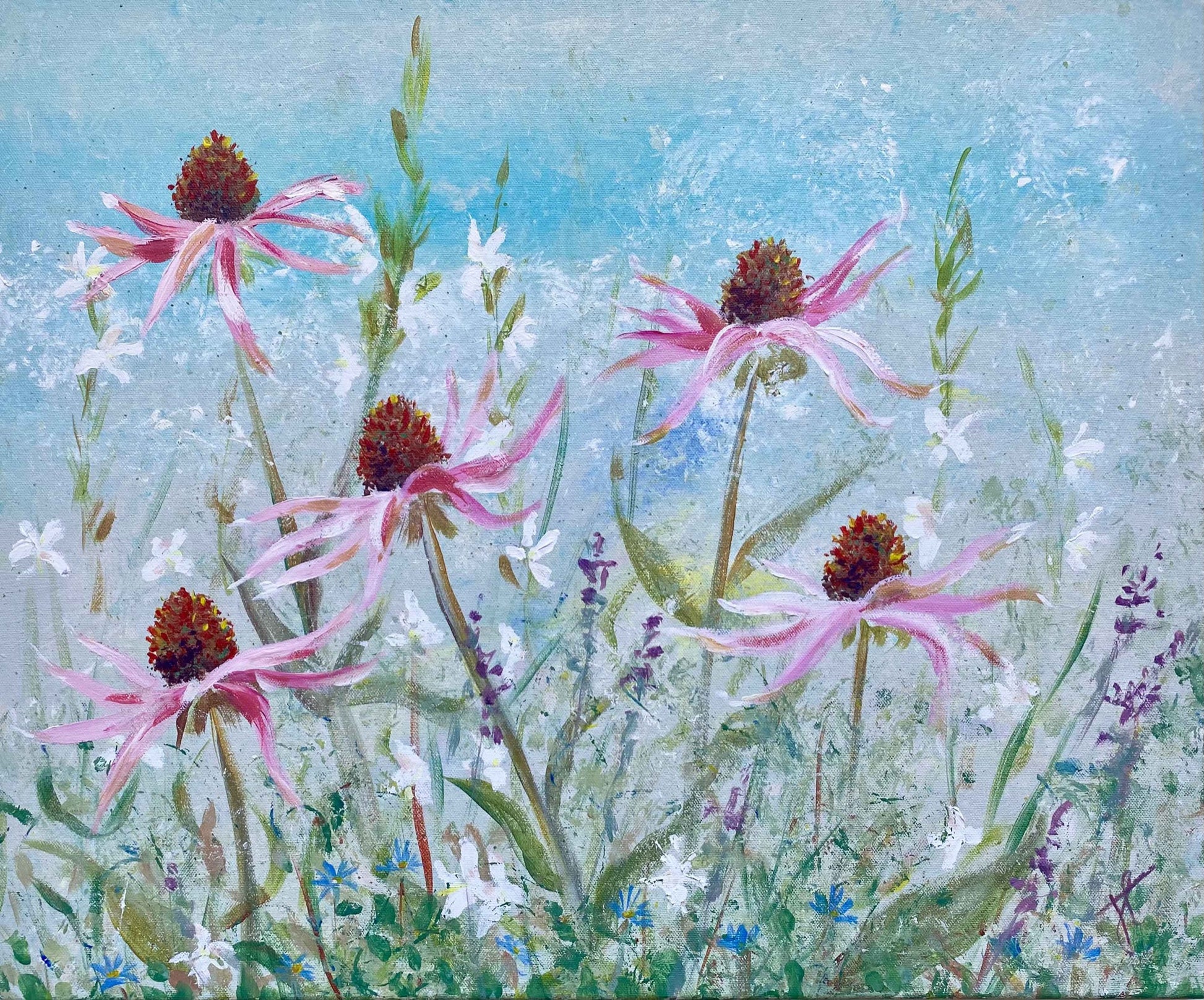This is a detailed watercolor painting featuring a vibrant garden scene against a blue and white sky, evoking a sense of the open, vast atmosphere. The foreground is dominated by large, vividly pink flowers with starfish-like pointy petals and round, reddish-brown centers. Scattered amongst the larger flowers are teeny tiny white flowers, all connected by green stems and leaves. Lower in the painting, near the base, are various smaller blooms: tiny blue flowers, petite purple flowers, and a row of very small purple flowers with dark green leaves. Additionally, there’s greenery throughout the painting, including lighter green leaves and other plants. The overall effect is a rich, colorful variety of flora set against a calming, sky-like backdrop.